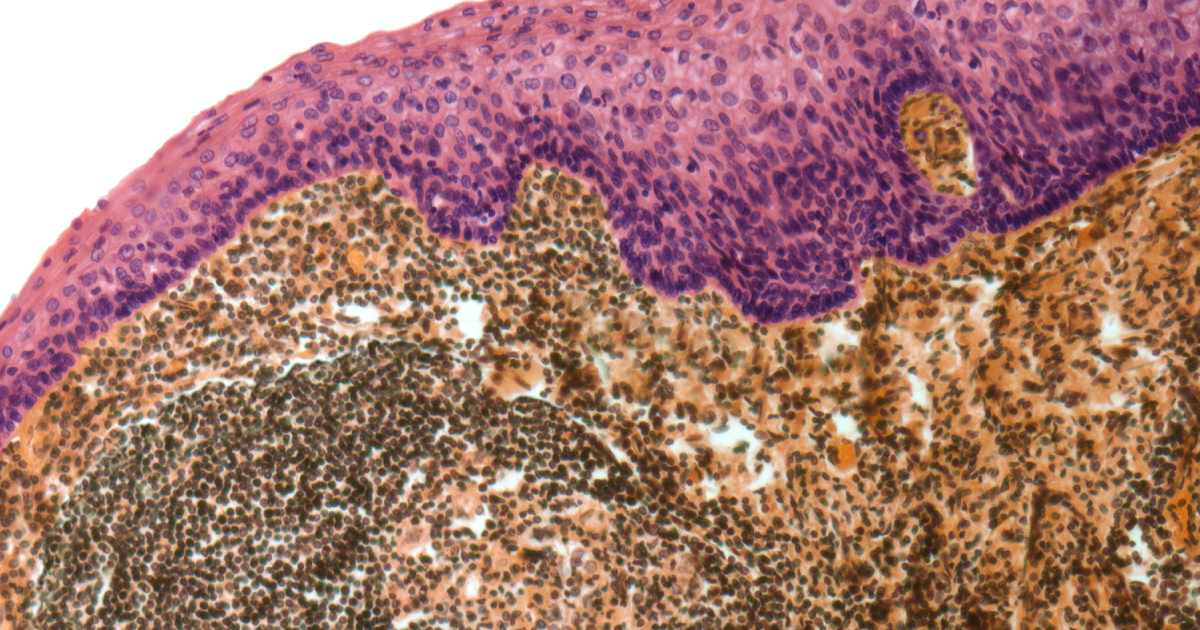This image portrays a highly magnified biological entity, primarily revealing a cellular structure. The photograph, in landscape orientation, showcases a dynamic interplay of colors and textures. Dominating the upper portion of the image is a vivid purple layer stained for visualization purposes, with a darker purple fringe concentrating around the center. The purple region gently slopes from the top right to mid-left, set against a pinkish backdrop. Below, the predominant light brown expanse features white speckles interspersed with denser black areas, possibly indicating different cellular components or concentrations. The cellular mass at the bottom includes dark brown and light brown cells mixed with sporadic white patches. The entire image is set against a stark white background, particularly blank in the upper left corner. This microscopic view, possibly a representation of human immune system tissue, blends scientific detail with illustrative precision, presenting a complex, grainy landscape of brown and purple hues devoid of any textual or illustrative annotations.